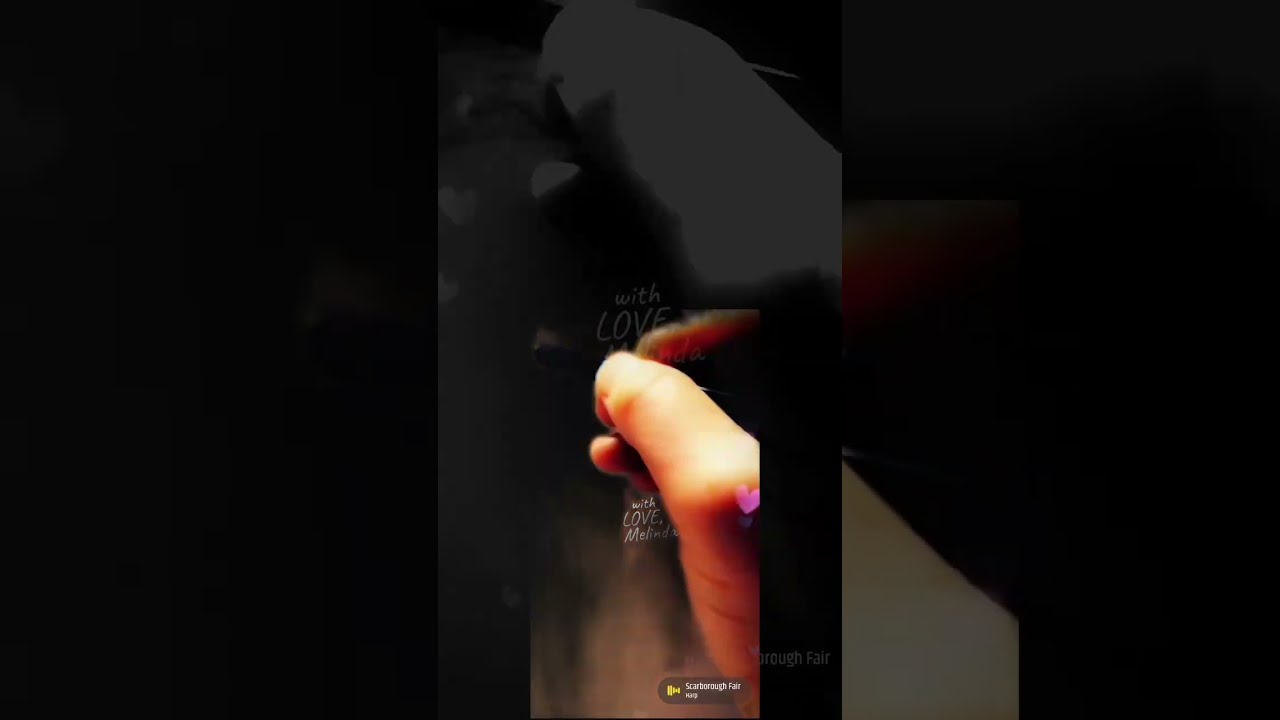The image features a tightly cropped view of a Caucasian person's right hand, with the thumb touching the index finger, forming a loose fist-like shape. The background is predominantly black, with the darkness consuming the left and right sides of the picture. At the center, the illuminated fingers are holding or touching what appears to be a piece of glass or an engraved steel surface. Above the thumb, there’s a small, pink cartoon heart. Below the fingers, in a delicate, seemingly hand-drawn white font, the inscription "With Love, Melinda" is visible, though somewhat obscured by reflections and blurriness. The background also contains an abstract, grayscale photo-negative-like mirroring of the hand, further adding to the image’s dark and intricate composition. The very bottom of the frame has small, indiscernible white text, adding an additional layer of detail to this enigmatic and reflective scene.